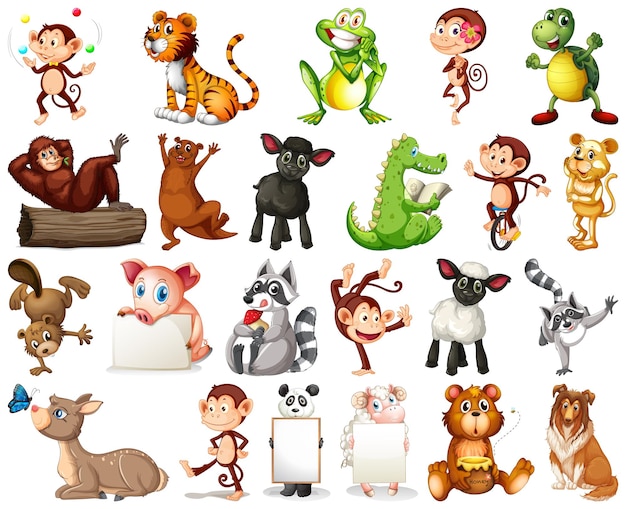This whimsical collection of vibrant clipart animals is set against a pure white background, organized into four rows, each brimming with animated figures in playful poses. In the top row, there is a smiley monkey juggling joyfully, followed by a tiger and a frog that seems to be eagerly awaiting something as it holds its hands in anticipation. A charming monkey with a flower tucked behind its ear gazes at the viewer, while a turtle, sporting red shoes, cheers energetically.

The second row presents an intriguing ensemble, beginning with an ape or chimpanzee resting slightly above a log. An otter-like creature reaches its arms skyward next to a playful black lamb. There is also a dragon engrossed in a book, a monkey balancing skillfully on a unicycle, and a lioness appearing thoughtful as it rests its cheek on one paw.

The third row showcases some impressive physical feats—a beaver executes a one-handed handstand, and next to it, a pig holds a blank white rectangle, presumably for personalization. Continuing the playful theme, a raccoon with its tongue sticking out holds a mushroom, while another monkey performs another one-handed handstand identical to the beaver's. A white sheep mirrors the black lamb from the previous row, and another raccoon does a handstand.

In the final row, a deer lounges gracefully while observing a blue butterfly. A casually walking monkey, a panda with a large blank white rectangle, and a ram each hold a similar blank rectangle for customizable messages. A bear, looking surprised, sits with a honeypot and a bee buzzing around it, while a border collie gazes warmly at the viewer.

This captivating ensemble of cartoon animals, richly detailed and colorfully illustrated, is perfect for delighting children with its varied and delightful characters.